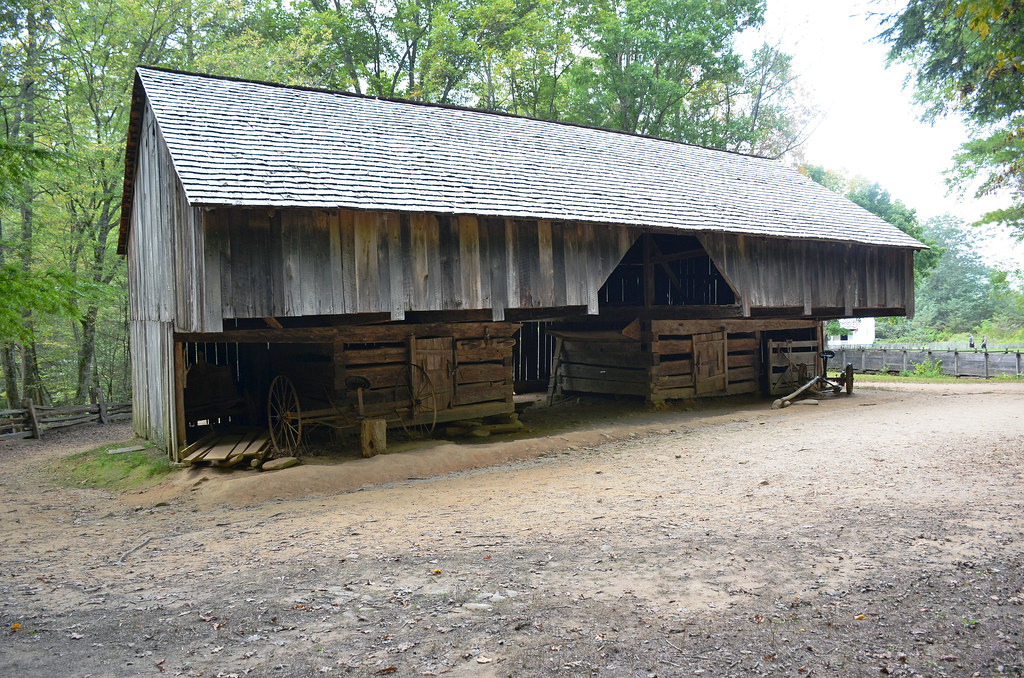This image depicts a long, rectangular, old barn settled on a dirt expanse with a rustic, rural ambiance. The barn's exterior features weathered gray boards covering the upper half, while the lower half reveals small animal pens constructed with medium-brown logs. These pens, located at the base, are equipped with doors, and a walk-through passage separates them, indicating a design likely intended for the care of animals. The barn's roof is steeply pointed and covered with shingled wooden tiles.

To the right of the barn, there is a wooden fence, and partially visible in the background is a white building, adding to the picturesque countryside setting. The environment around the barn is mostly dirt with some hints of green vegetation towards the left side of the image. The backdrop is filled with trees, and the sky appears bright white towards the upper right, enhancing the sense of an open and airy rural landscape. Notably, in front of the pen on the left side of the barn, two wagon wheels are situated, adding further to the scene's historical charm and rustic appeal.